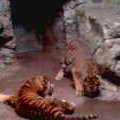The image depicts two tigers inside an enclosure with mock natural features resembling a rocky cave. The photograph is small, blurry, and out of focus, making it difficult to discern clear details. The enclosure's floor has a dark brown-red hue. One tiger lies on the ground facing away from the camera, with one paw extended to the left and the other underneath, its legs spread to the right, and its tail down. Adjacent to this tiger, another appears to be standing with its head facing downward, possibly eating, although the image quality makes it challenging to be certain. The background includes a large stone piece on the right and an opening in the stone wall, reinforcing the cave-like setting.